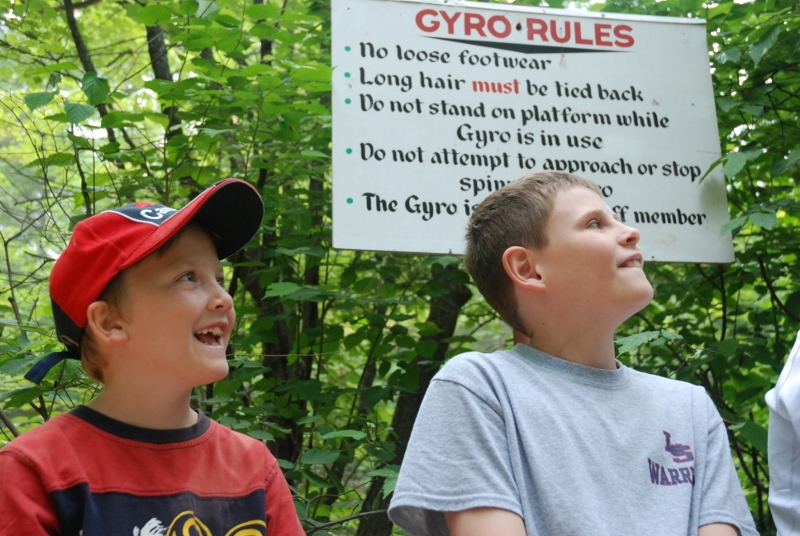In this photo, two boys are captured in a woodland setting, emphasized by the solid tree line behind them. Both boys are looking upward to their right with expressions of anticipation and excitement. The boy on the left is sporting a red baseball cap with a black front and white writing, paired with a red shirt featuring a black front. The boy on the right is in a gray t-shirt with blue writing. To his left, which is our right, there's an obscured individual whose shoulder is barely visible.

Behind the boys hangs a poster affixed to a tree, displaying a large red header that reads "Gyro Rules." This sign includes a bulleted list of instructions for using a gyro, stating: "No loose footwear," "Long hair must be tied back," "Do not stand on platform while gyro is in use," "Do not attempt to approach or stop spinning gyro," and a partially obscured fifth rule.